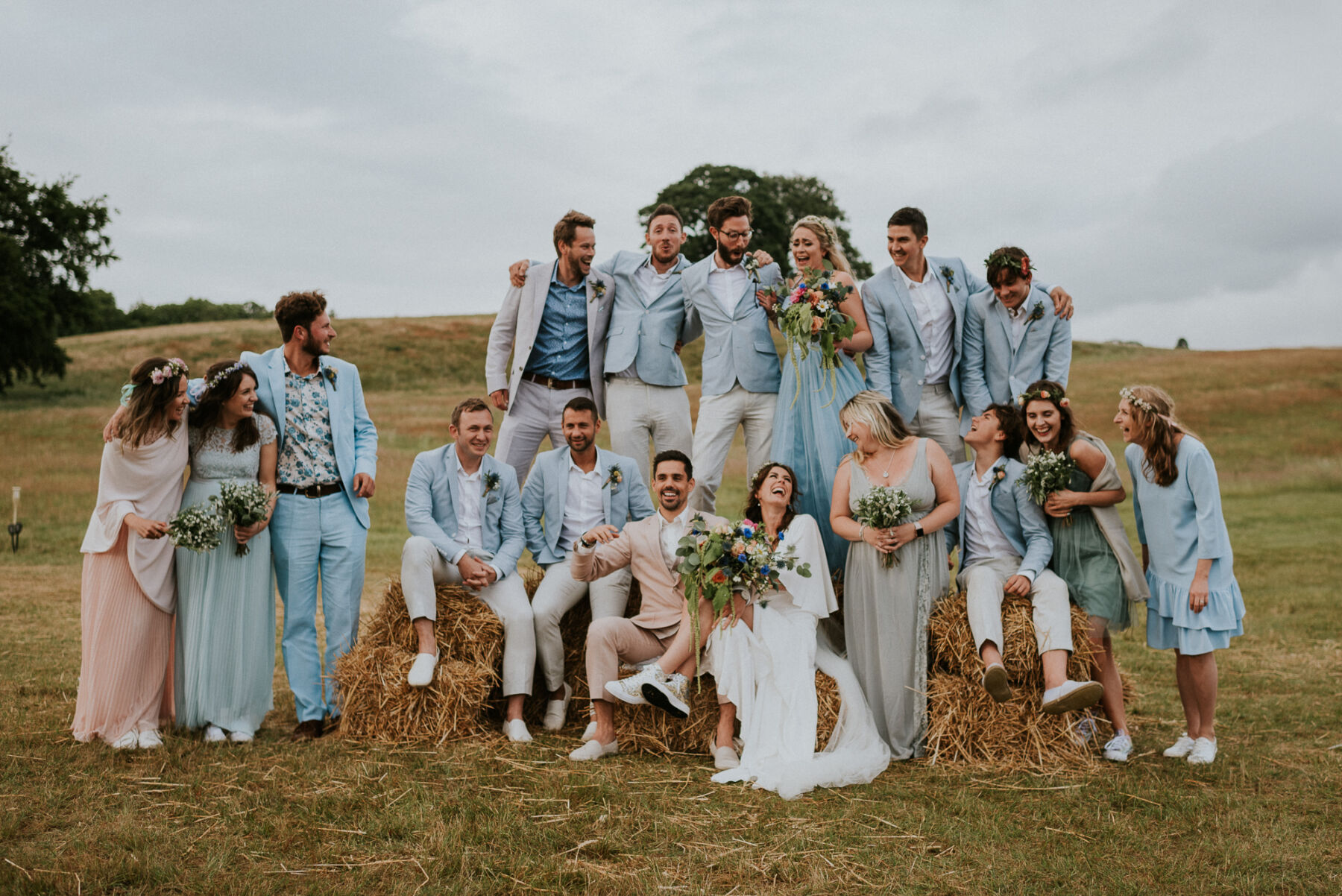This photorealistic image captures an outdoor wedding scene, featuring a joyful party of 17 people perched on hay bales set in a sprawling, hilly meadow under a cloudy, hazy sky. Two brides, glowing in long, swooping white dresses, and two grooms, one notably in a pale pink tuxedo, are front and center, surrounded by bridesmaids and groomsmen dressed in light, pastel colors—blues, pinks, grays, and peach. The party, including women ranging from the bride to the matron and maid of honor, all carry flowers and exude happiness through their bright smiles and laughter. The grassy field, tinged with hints of an approaching fall, is accented by a couple of scattered trees, enhancing the serene, rustic charm of the setting. The group, all appearing to be no older than their early 30s, embodies a radiant, youthful exuberance in this seemingly double wedding celebration.